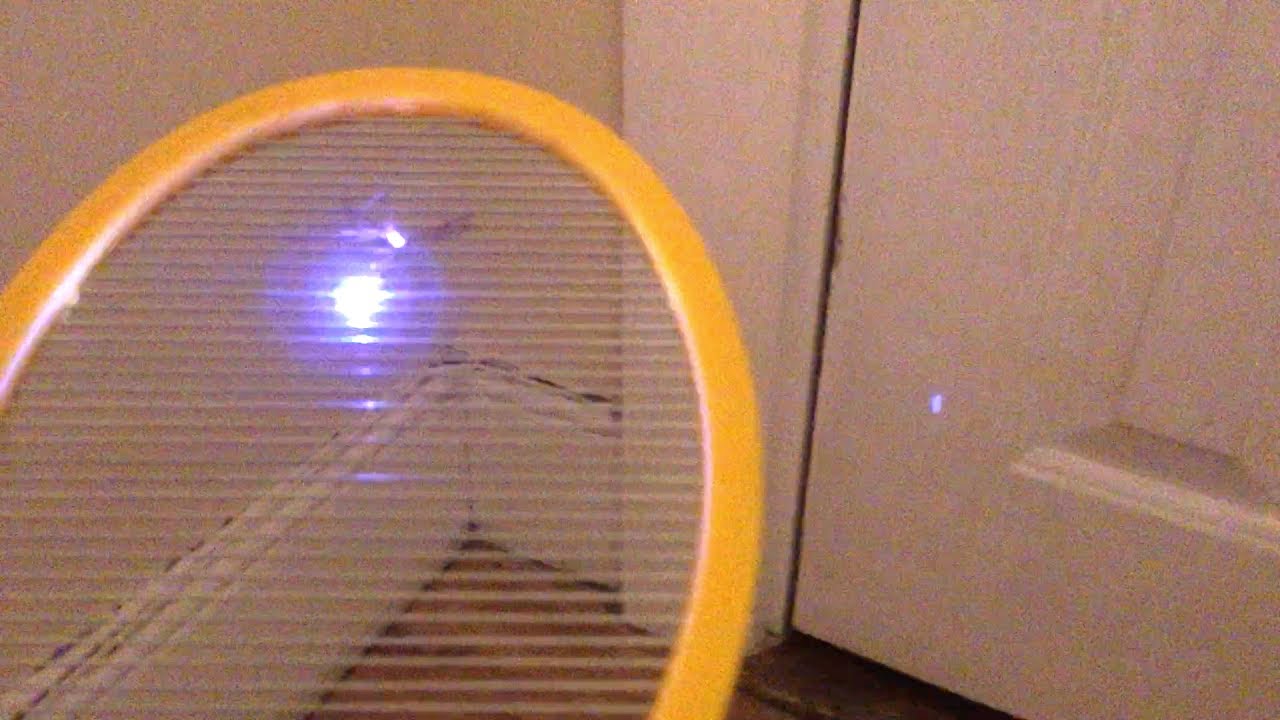The photograph depicts a person holding an electric fly swatter with yellow edges, actively zapping a bug. The mesh of the swatter is illuminated with a striking blue spark, capturing the moment of electricity hitting the bug. The background reveals an older or poorly maintained room corner, characterized by beige walls, white baseboards, and door trim, as well as a white-framed door. On the floor, the worn tan to light brown wood adds to the room's vintage feel. A wicker chair appears in the frame, providing a glimpse through to the purple and blue glow, likely caused by the camera flash. The detailed scene is set against this intricate, slightly dilapidated interior, emphasizing the bright zap of the fly swatter against the otherwise subdued setting.